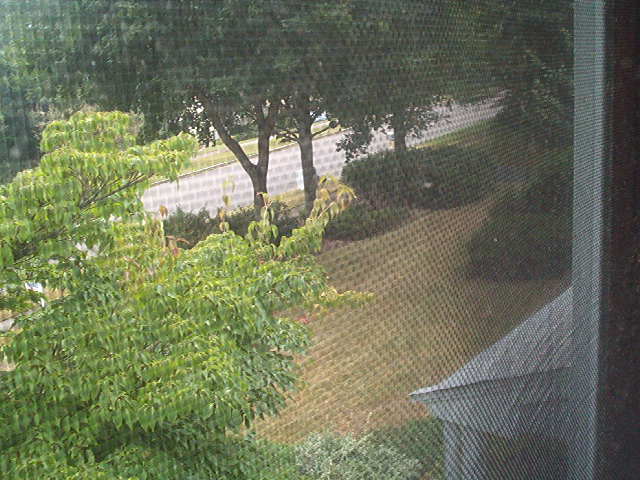This photograph, taken from inside a building through a soft mesh or window screen, captures a detailed view of a front yard, likely of a home. The perspective is from an upper floor, looking down at the landscape below. Dominating the foreground is a green tree situated close to the mesh. Beyond this tree, the yard features several more trees, each with neatly landscaped bushes at their bases. 

The grass appears worn or partially brown, possibly indicating a dirt driveway, leading to a simple tree-lined street. Hedgerows and various trimmed plants add structure and greenery to the scene. On the far side of the yard, past the trees, a paved road can be seen, along with hints of another house visible through the foliage. 

Notably, the bottom right corner of the photo shows part of a white-covered porch or balcony of the viewed home, supported by dual pillars. This detail suggests an inviting and well-maintained entryway to the property. The entire image conveys a sense of tranquility, blending natural elements with residential architecture.